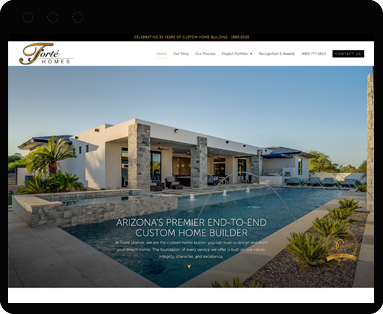A screenshot of a website is displayed on a tablet, featuring a sleek black navigation bar at the top with minuscule, illegible text. Below, a white banner prominently showcases "Forte Holmes" with an elegant 'F', positioned in the upper left corner. The navigation menu includes clickable options such as "Home," "Our Story," and potentially "Our Store," among other indistinct gray links against the white background. To the right of the menu is a search bar.

Beneath the banner, an image of an opulent, architecturally unique home is showcased. Described as both a modern factory and a Mexican villa, the house features squared architecture, with gray stone pillars that contrast sharply with its tan stucco-like exterior. Expansive glass windows dominate the front facade, offering views of a finely-crafted swimming pool with steps leading into the water, suggesting it is meant for use rather than merely for decoration. The surrounding desert landscape enhances the luxurious feel of the property, with carefully selected plants and vegetation.

The website highlights its status as "Arizona's premier end-to-end custom home builder," implying that such bespoke homes come with a substantial price tag. The overall design and content suggest a focus on high-end, custom-built homes tailored to affluent clients in a desert setting.